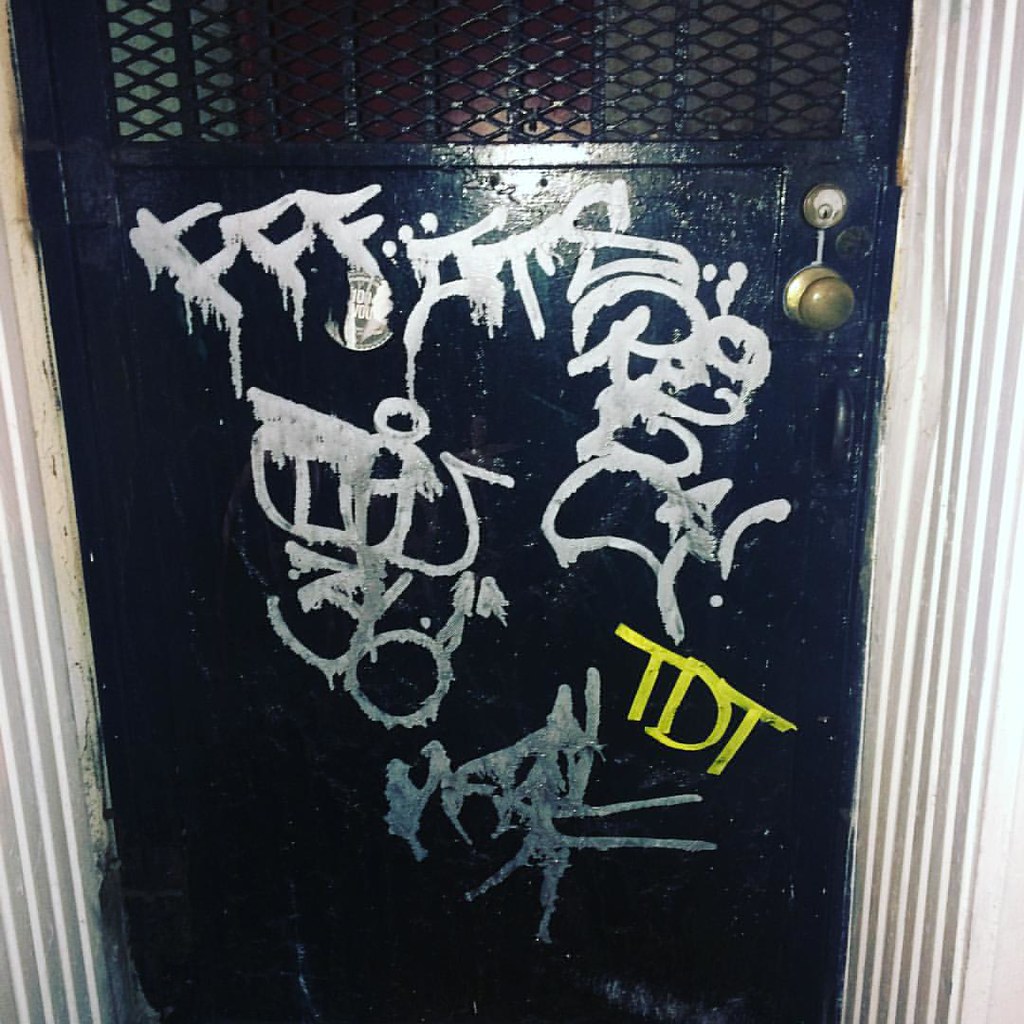This photograph captures the lower half of a black door, which appears to be either painted wood or metal, framed by a white, bumpy, wooden or aluminum trim. The door features a silver doorknob and a lock situated just above it. Higher up, there is a hole cut in the door, fitted with a tight metal mesh screen. Graffiti in various colors, primarily gray and white with notable patches in bright yellow, covers the middle section of the door. Among the graffiti are the characters "FFF," the number "36," and the initials "TDT." The white paint of the graffiti is dripping and adds to the overall chaotic appearance. Adjacent to the door, the wall is adorned with long vertical stripes in gray and white. The black paint on the door is high-gloss, reflecting light from an unseen source. The overall scene has a raw, urban aesthetic, marked by the poorly executed paint job that bleeds onto the frame.